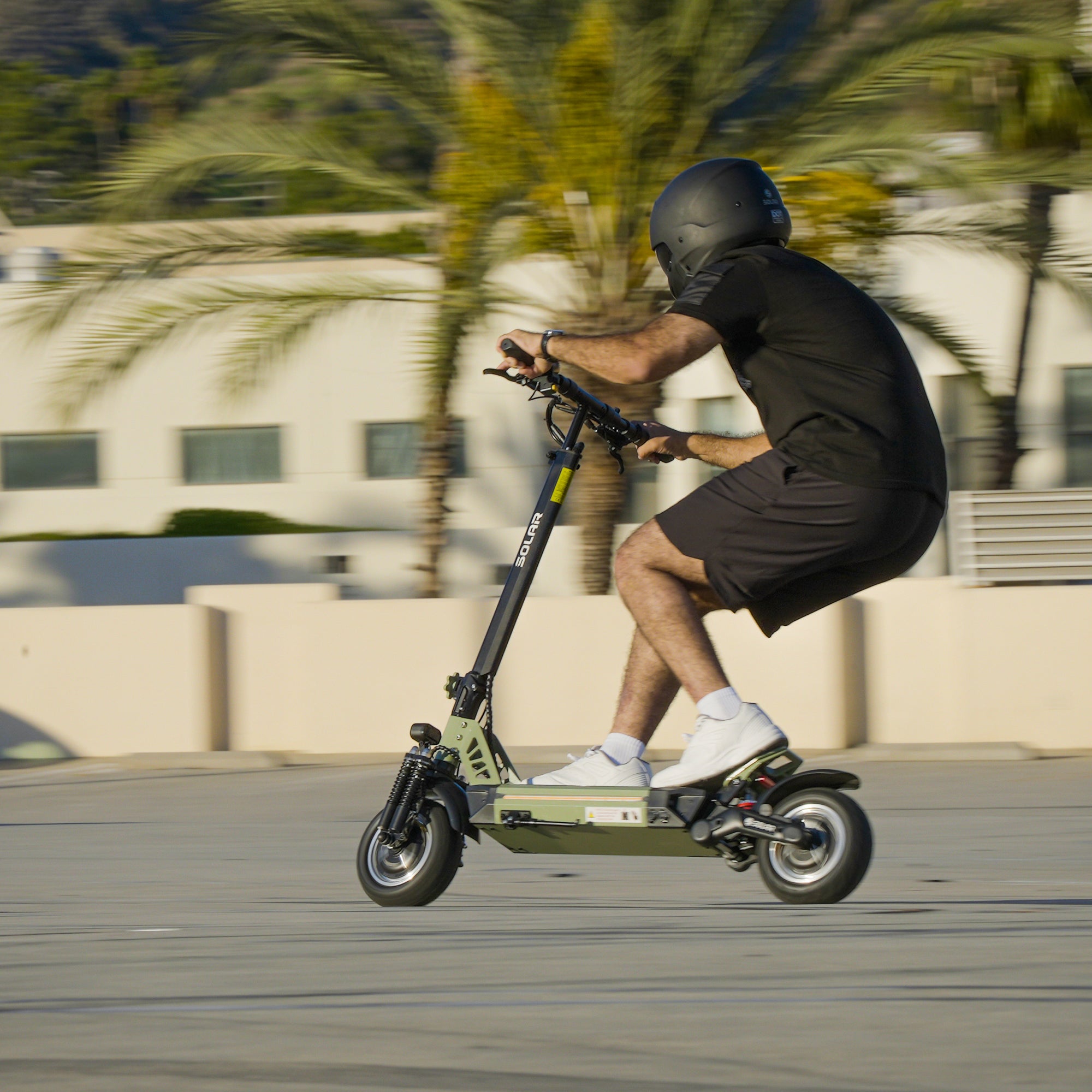This vivid color photograph captures an action shot of a young man riding an olive green scooter. The scooter, likely battery-powered, features black metal components, rubber pneumatic tires, and possibly a disc brake. The rider, clad in a black helmet reminiscent of Darth Vader's, a black t-shirt, black shorts, and white socks and sneakers, is in profile. His legs are positioned with one foot centrally on the scooter and the other extended back, indicating swift motion. The scooter boasts a black bar marked with "Flyer" or "Solar" in white letters. The backdrop is a heavily blurred scene, enhancing the sense of speed, featuring a white stucco building with multiple windows and green palm trees, all set against a tan setting. The man’s bent posture and raised arms gripping the flat handlebars contribute to the dynamic feel of this well-composed shot.